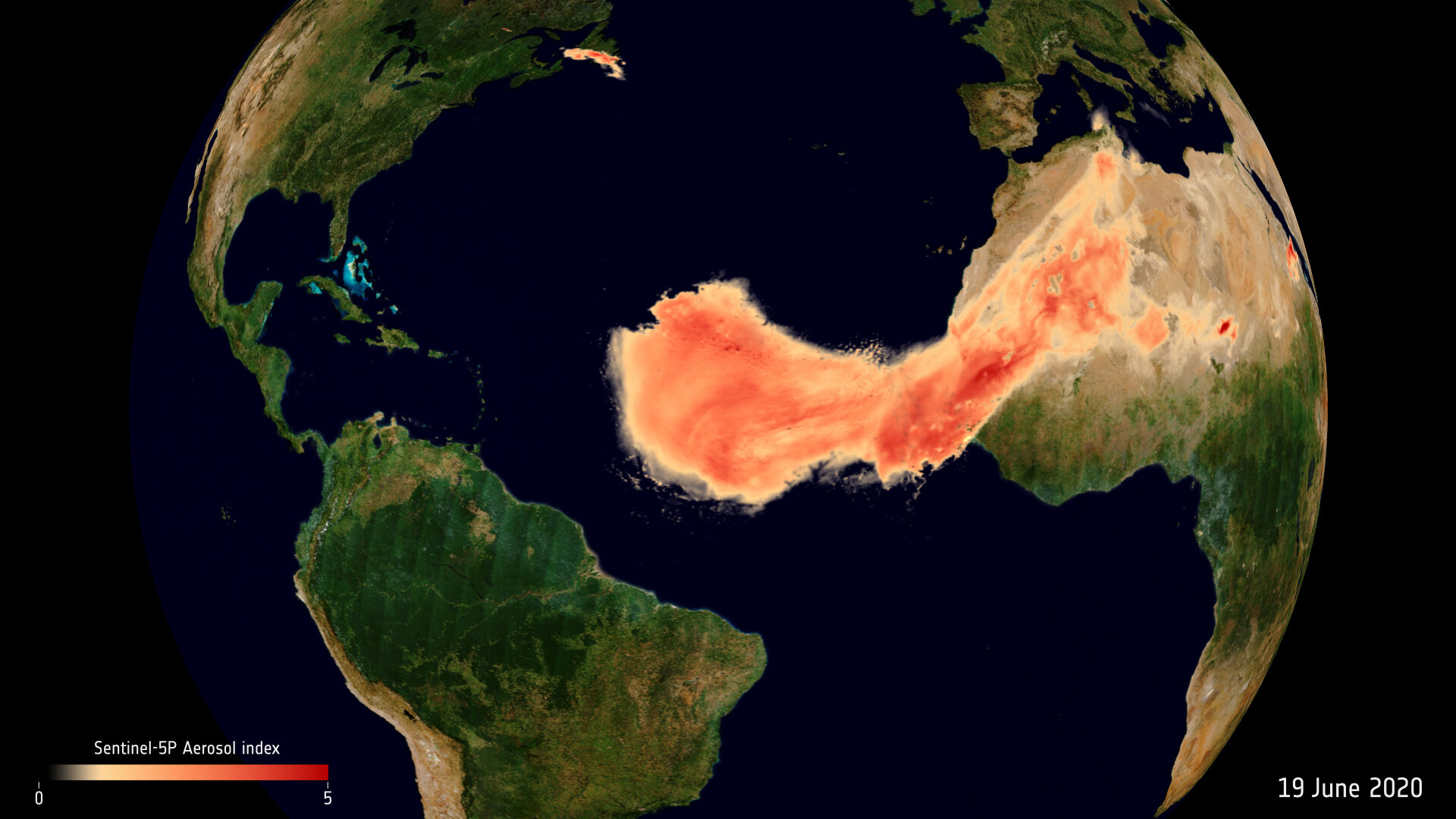This photograph, seemingly taken from space, captures the Earth with a striking portrayal of its continents and an evident focus on atmospheric phenomena. The image features a dark background speckled with white dots, representing stars. In the foreground, Earth is depicted in a dark blue hue, almost blending into the blackness of space. The continents are distinctly visible in green and tan shades, with the United States and the Americas on the left and Africa and Europe on the right.

Dominating the Atlantic Ocean, a large, multicolored cloud in shades of red, orange, and yellow signifies significant aerosol pollution—potentially a dust or sand cloud from the Sahara Desert. This vivid feature illustrates the extent of the aerosol dispersion. Small printed text at the bottom left corner reads "Sentinel-5P Aerosol Index," referencing the satellite responsible for the data collection, with a color scale indicating varying pollutant levels, where zero is yellow and five is red. On the bottom right, the date "19 June 2020" is displayed, grounding the observation in a specific temporal context.